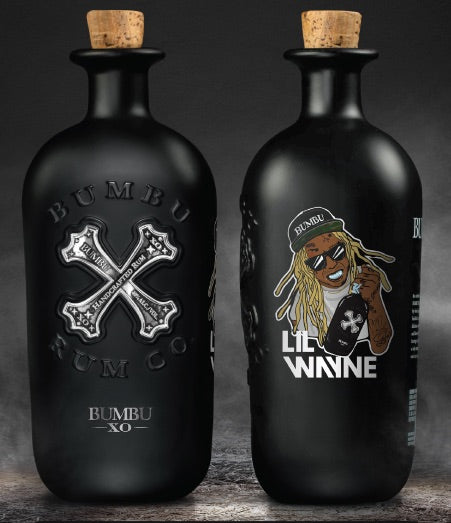The image features two black bottles with wood corks set against a smoky gray background. The bottles, completely matte black and opaque, are prominently displayed in the foreground. The photograph is cleverly split down the middle, perfectly separating the two bottles. The bottle on the left displays the front view which showcases "Bamboo Rum Co" in raised lettering. At the center, a silver "X" is displayed with the phrase "Handcrafted Rum" diagonally inscribed from the bottom left to the top right. At the bottom of the bottle, "Bamboo XO" is written in silver text. On the right side of the image is the back view of the bottle, featuring a stylized cartoon illustration of Lil Wayne. He is depicted with yellow-golden dreadlocks, wearing black shades, and a black baseball hat that reads "Bamboo" in white letters. Lil Wayne is shown holding the same bottle, with his name written in white font underneath the illustration.